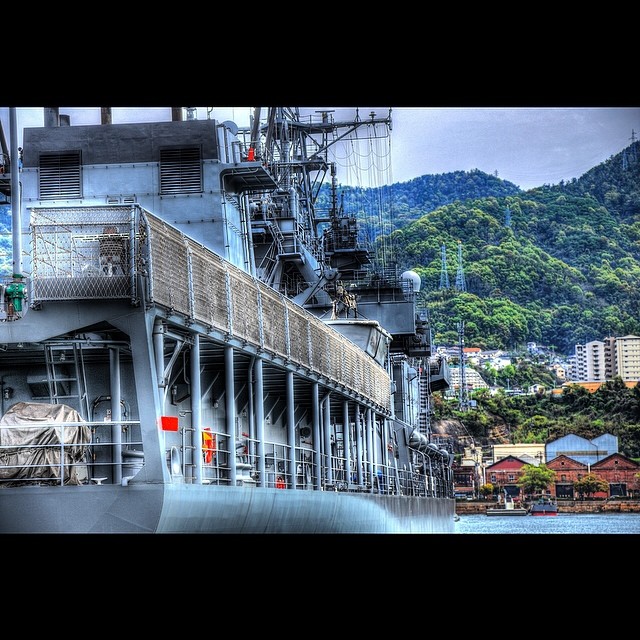In the foreground, the image captures a ship with multiple decks: a top deck, a bottom deck, and an additional upper deck. The ship is encircled by guard rails that resemble chain link fences, likely designed for safety and to facilitate the loading and unloading of cargo. The vessel is equipped with various apparatus, probably used for handling goods. 

In the background, a bustling dock can be seen, populated with a few more ships and a cluster of buildings that presumably serve the dock workers. These structures are dwarfed by taller buildings further back, which blend with the backdrop of a magnificent mountain range covered in dense forests. The overall sky above the scene is a serene light blue.

The color palette in the image includes hues of light blue, chain link gray, various shades of greens, vibrant reds, light yellow, and forest green, creating a visually striking composition. The setting appears to be either by the sea or a large lake adjacent to a forest, culminating at a busy dock.